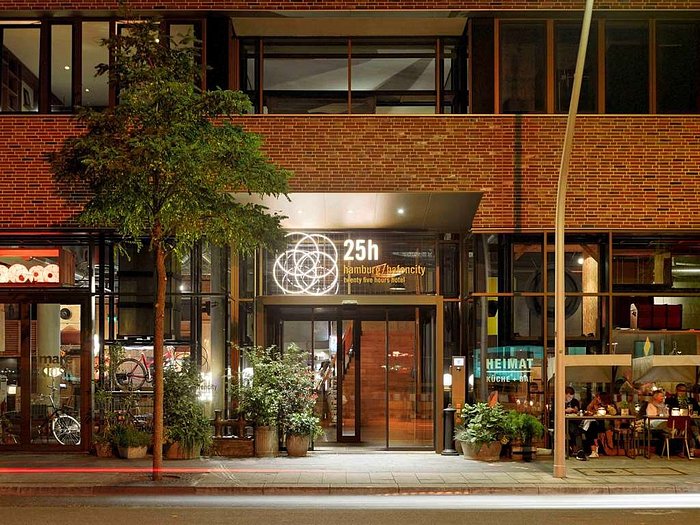The photograph captures the front of a multi-storey brick building, likely taken from the opposite side of a well-illuminated street at nighttime. The ground floor features a series of large windows and transparent surfaces, alongside a restaurant or storefront named "25H Hemberg / Benefactory." The sign, positioned above a glass entrance door, is partially obscured, with smaller unreadable text due to the bright street lights. Flanking the doorway are several potted plants. To the left, a bike shop with numerous bicycles inside can be seen. The upper levels showcase expansive glass windows set within a brown brick facade. The scene includes additional details such as a streetlight pole, trees lining the pavement, and small kiosks with tables where people are seen selling items. There’s also a sitting area outside another shop where people are dining, enhancing the lively nighttime atmosphere.